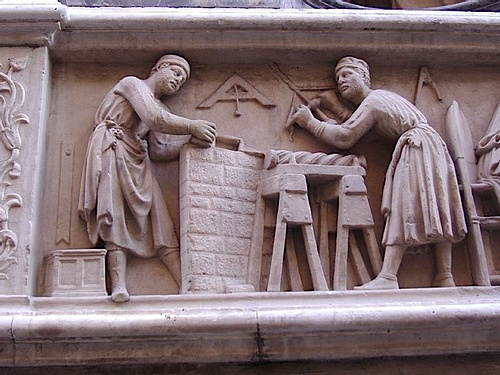The photograph depicts a detailed stone sculpture set into a natural-lit, horizontally rectangular frame devoid of any borders or background. In this 16th-century styled artwork, two men, dressed in robes cinched with belts and wearing shoes, are depicted as artisans engrossed in their craft. 

The man on the left stands over a light brown or beige brick wall, handling blocks of brick with old-fashioned tools scattered nearby. To his side lies a cubic box and above his head, a large letter "A" combined with a small swinging bell suggests the presence of a clock. The other man, positioned on the right, works over a pair of wooden sawhorses, interacting with what looks like a piece involving a triangle and a stick. He is surrounded by additional metalworking tools and a wooden shelf.

Both figures are positioned within an intricately decorated stone framework featuring vertical stone pillars with triangular peaks, adding to the historical ambiance of the scene. The overall texture and hue of the sculpture appear in light brown tones, emphasizing the artistic finesse of this stone depiction of two dedicated craftsmen.